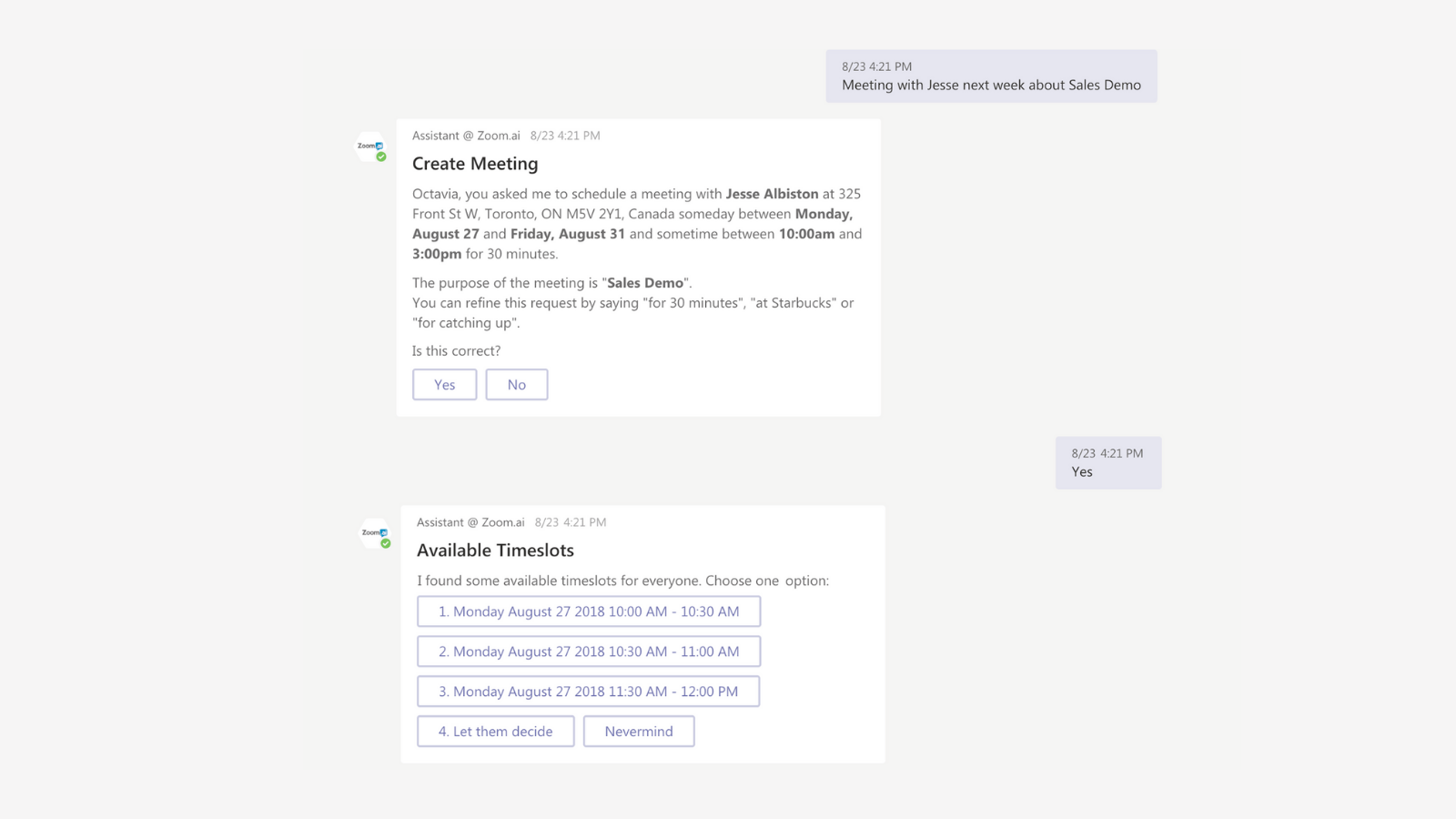Here is a cleaned-up and detailed descriptive caption based on the voice input provided:

---

The screenshot displays a scheduling interface for creating a meeting. The top section of the interface prominently features the header "Create Meeting." Below this, there are options to confirm or deny the meeting creation, indicated by "Yes" or "No" prompts. There is a field where the meeting details can be entered, though it is not filled in this instance. 

Following this section is a list of available time slots. Each time slot is accompanied by a small icon that is too small to decipher, likely indicative of a collaborative tool or platform. The available time slots for Monday, August 27 are as follows:
- 10:30 AM to 11:00 AM
- 11:00 AM to 11:30 AM
- 12:00 PM to 12:30 PM

Additional text within the interface suggests options for allowing participants to decide the time or canceling the meeting. There’s also a text message conversation element, where one of the messages mentions a meeting with someone named Jesse next week. 

The overall design and organization of the interface appear to involve components of both a scheduling application and a messaging platform, facilitating streamlined meeting coordination.

---